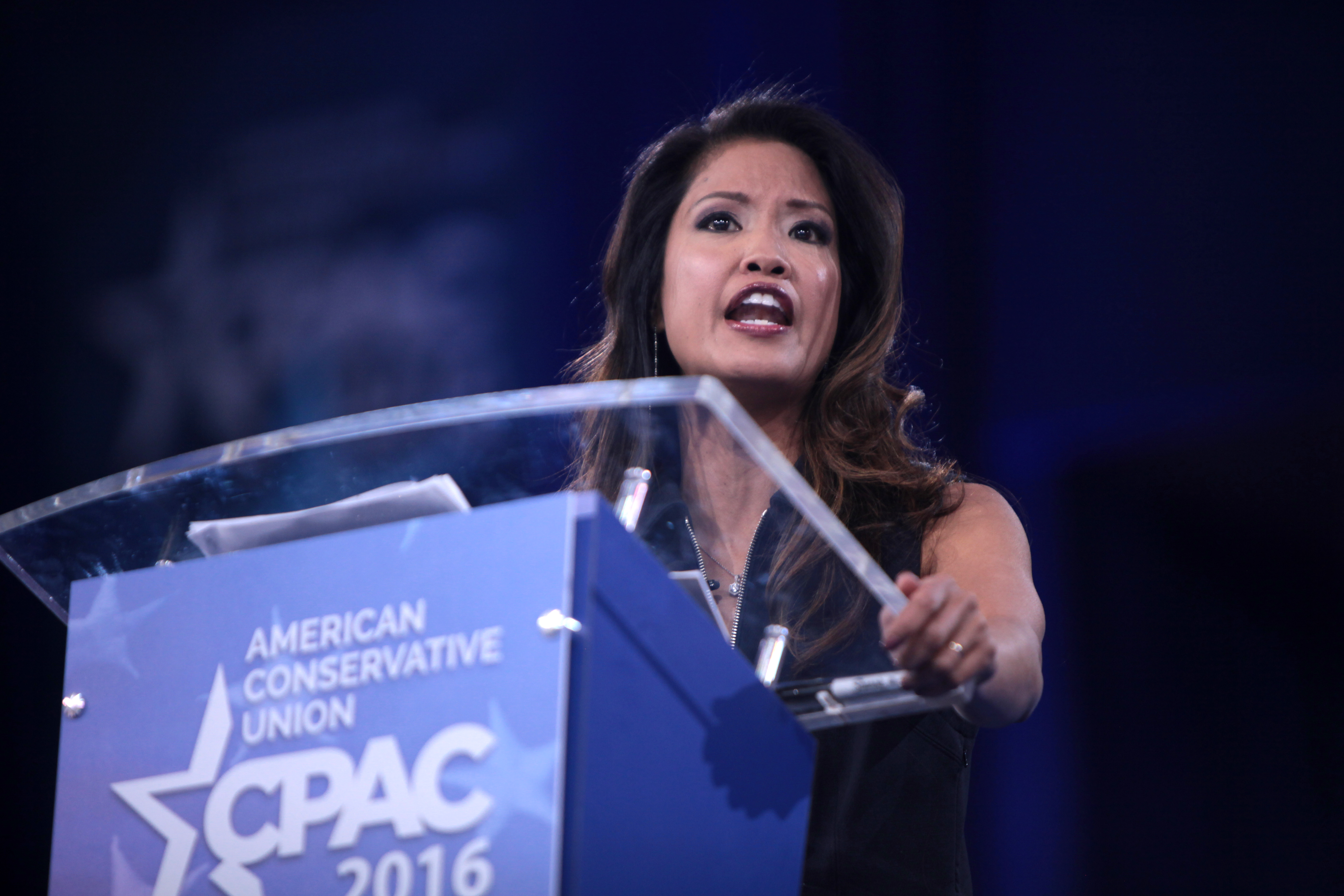This image captures a vibrant indoor scene at a conference, likely CPAC 2016, organized by the American Conservative Union. The background is awash in dark blue hues with hints of black, featuring some blurred white writing and possibly a curtain or banner in blue tones. Dominating the left-hand foreground is a blue podium with a distinctive plexiglass top. Emblazoned in white text on the podium are the words "American Conservative Union," accompanied by a half-star logo and "CPAC 2016."

Behind the podium stands a poised lady of apparent East Asian descent, delivering a speech. She has long, dark brown hair styled in loose waves cascading around her shoulders. Her outfit consists of a sleeveless, black top partially unzipped to reveal a pearl necklace. Her lips are painted dark red, and she speaks with her mouth open, showing both her upper and lower teeth. Her dark eyes convey focus as she looks into the distance. One of her hands grips the plexiglass overhang of the podium, adorned with a gold ring on her ring finger. The photo, measuring approximately six inches wide and four inches tall, offers an upward perspective of her, emphasizing her engagement and the event’s atmosphere.